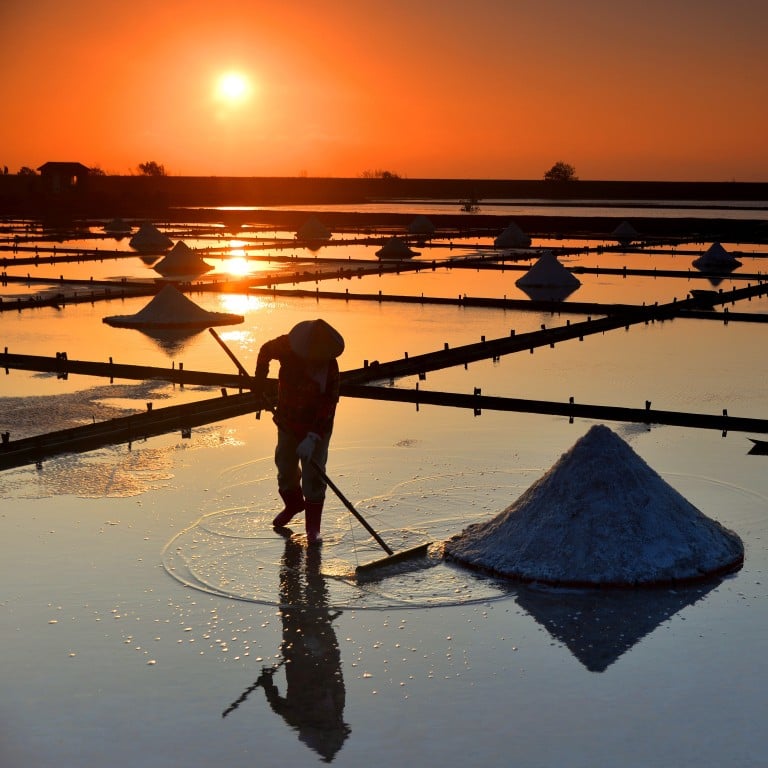The image depicts a serene Asian landscape featuring expansive rice paddies under a low, orange-tinted sun. The sky glows warmly, hinting at either sunrise or sunset, and trees grace the distant background. A man is at the center, wearing an iconic Asian conical hat that shades his face. Dressed in practical boots for wading through the shallow, reflective water, he wields a large push broom. He's methodically gathering and sweeping the contents of the water into neat, pyramid-shaped piles, identifiable as salt. Each square pool around him mirrors both the sky and the accumulated piles of salt, indicating a methodical salt-harvesting process. The man’s silhouette is mirrored in the glistening pools, adding to the picturesque quality of the scene.